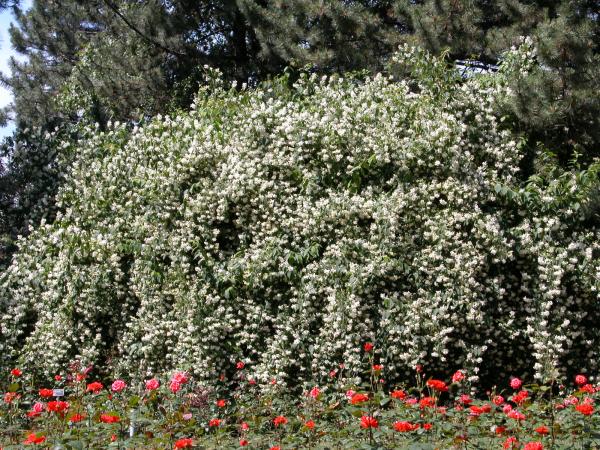This outdoor daytime photograph beautifully captures a vibrant and lush scene dominated by various plant growths. In the foreground, a mix of red and pink roses stands out, their colors bright against a backdrop of green stems and a hint of grass. Moving to the middle section, the scene is overtaken by a sprawling, dense bush or short tree heavily adorned with green leaves and an abundance of small white flowers, creating a striking contrast that almost makes the plant appear more white than green. The top section of the image is framed by tall evergreen or pine trees, their branches and needles stretching into the sky. The light is strong, likely from a high noon sun, casting downward shadows and revealing patches of blue sky through the gaps in the trees. This composition culminates in a rich tapestry of botanical life, blending vibrant colors and lush greenery under the clear, bright daylight.